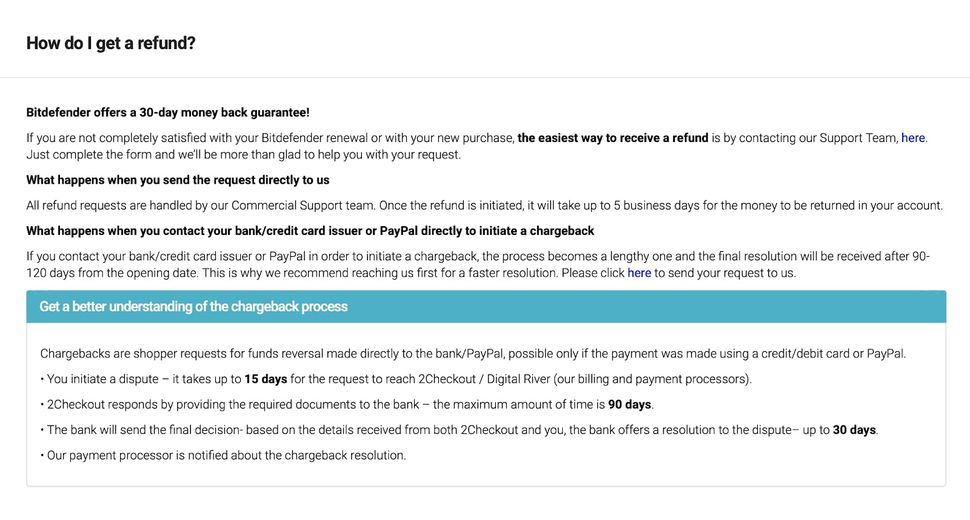**Detailed Caption:**

The image displays a webpage dedicated to refund procedures for a service called Blind Fender. At the top left corner, there is a prominently bolded heading in black font: "How do I get a refund?". Below this heading, in a moderately bolded font, it states, "Blind Fender offers a 30-day money-back guarantee". 

Following this, in standard, unbolded black font, a detailed description of the 30-day money-back guarantee is provided. Within this description, a key phrase "the easiest way to receive a refund" is emphasized in bold. A hyperlink labeled "here" is included, which directs users to contact support for refund assistance.

Further down, another bolded section title in black font reads: "What happens when you send a request directly to us?". This is followed by a descriptive sentence explaining the process of handling direct refund requests.

The third bolded question, "What happens when you contact your bank, credit card issuer, or PayPal directly to initiate a chargeback?", also appears in dark black font. This section includes another "please click here to send a request to us" hyperlink.

At the bottom of the page, there is a light blue, almost aqua-colored bar that instructs users to "Get a better understanding of the chargeback process". Below this bar, the text explains that chargebacks—requests for fund reversals—need to be directed to the bank or PayPal, and are possible only if the payment was made using a credit/debit card or PayPal. Four bullet points further elucidate this process.